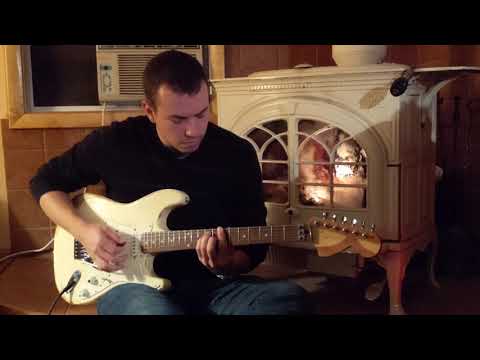In the image, a man with short dark hair and pronounced eyebrows is playing an electric guitar that is mostly white with cream accents. He is seated on a bench or chair, wearing blue jeans and a black long-sleeve shirt that reaches his elbows. His right hand is strumming the guitar while his left hand is positioned on the neck, searching for chords. The guitar is plugged in, with a cord running from its bottom, although its destination is unclear.

The background, partly overexposed and shadowy, features several distinct elements. To the man's left, there is a window-mounted air conditioner, and on his right, there is a fireplace with a glass door and an object sitting atop its mantle. Additionally, there is a white cabinet with short wooden legs and glass front doors, positioned near the fireplace. This cabinet supports a pot on its surface. The entire scene is framed by black borders at the top and bottom, giving the image a distinct, framed appearance.